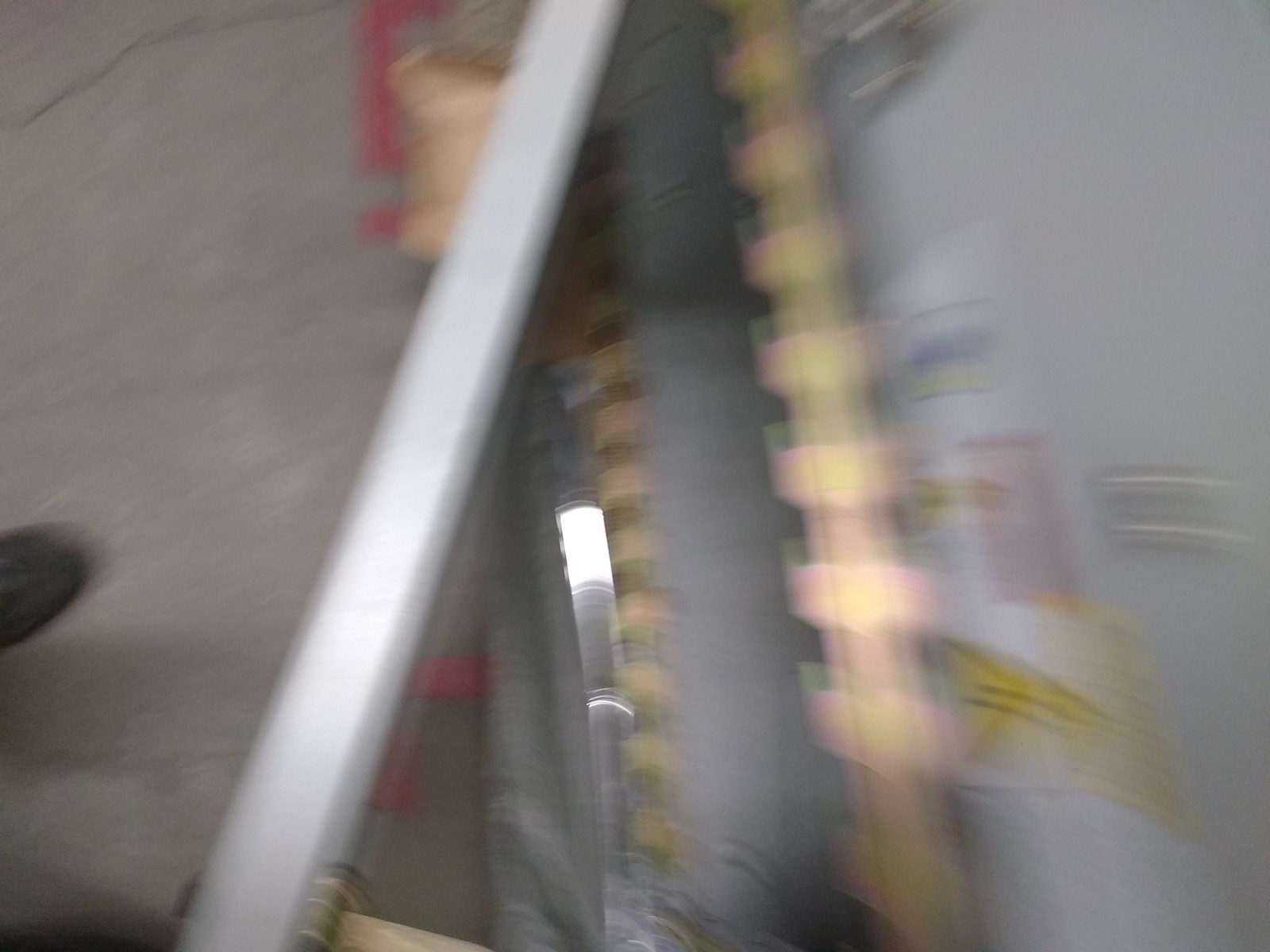This photograph features a highly blurred close-up of an object, making it challenging to discern specific details. The image appears to suffer from motion blur, particularly noticeable on the right side of the frame. On the left side, the blur is slightly less pronounced. Dominating the composition is an angular metal bar or piece that stretches diagonally from the top left to the bottom right at an approximate 30-degree angle. In contrast, another, potentially gold-tinted bar runs in a diagonal direction from the top right to the bottom left, intersecting the first bar at mid-frame. This gold-tinted bar has smaller protrusions or "little bars" along its length. Separating these two diagonal elements, a silver bar runs vertically through the middle, suggesting a structural component or connection between them. While it's difficult to conclusively identify the object, the arrangement of elements hints at a possible watch or clock mechanism.